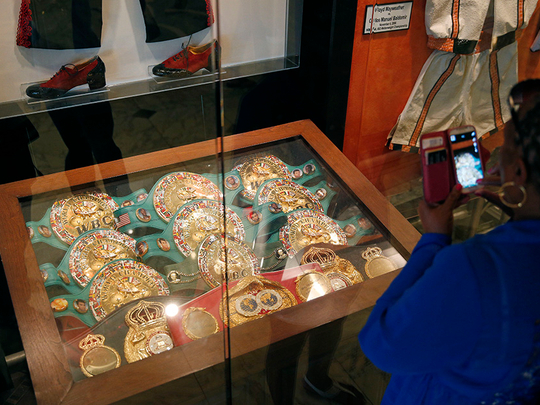In a vibrant museum setting, a black woman with short hair or an updo, adorned with gold hoop earrings, stands in the lower right corner, immersed in capturing the display with her phone, which has a red or pink purse-like cover containing credit cards. She is dressed in a royal blue dress or shirt. The centerpiece of the scene is a framed wooden display case with a glass front, showcasing various belts with large golden medallions. Predominantly, there are green bands with button-like designs and small faces, interspersed with a red band featuring a gold circle. Above the display, a pair of red and black shoes and matching pants are visible, set against a black backdrop with an open window. To the right of the main display, there's an outfit comprising white shorts with orange and black stripes alongside a matching jacket, against a red wall. The combination of these elements creates a rich tapestry of colors and textures, highlighting the intricate details and artifacts within the museum.